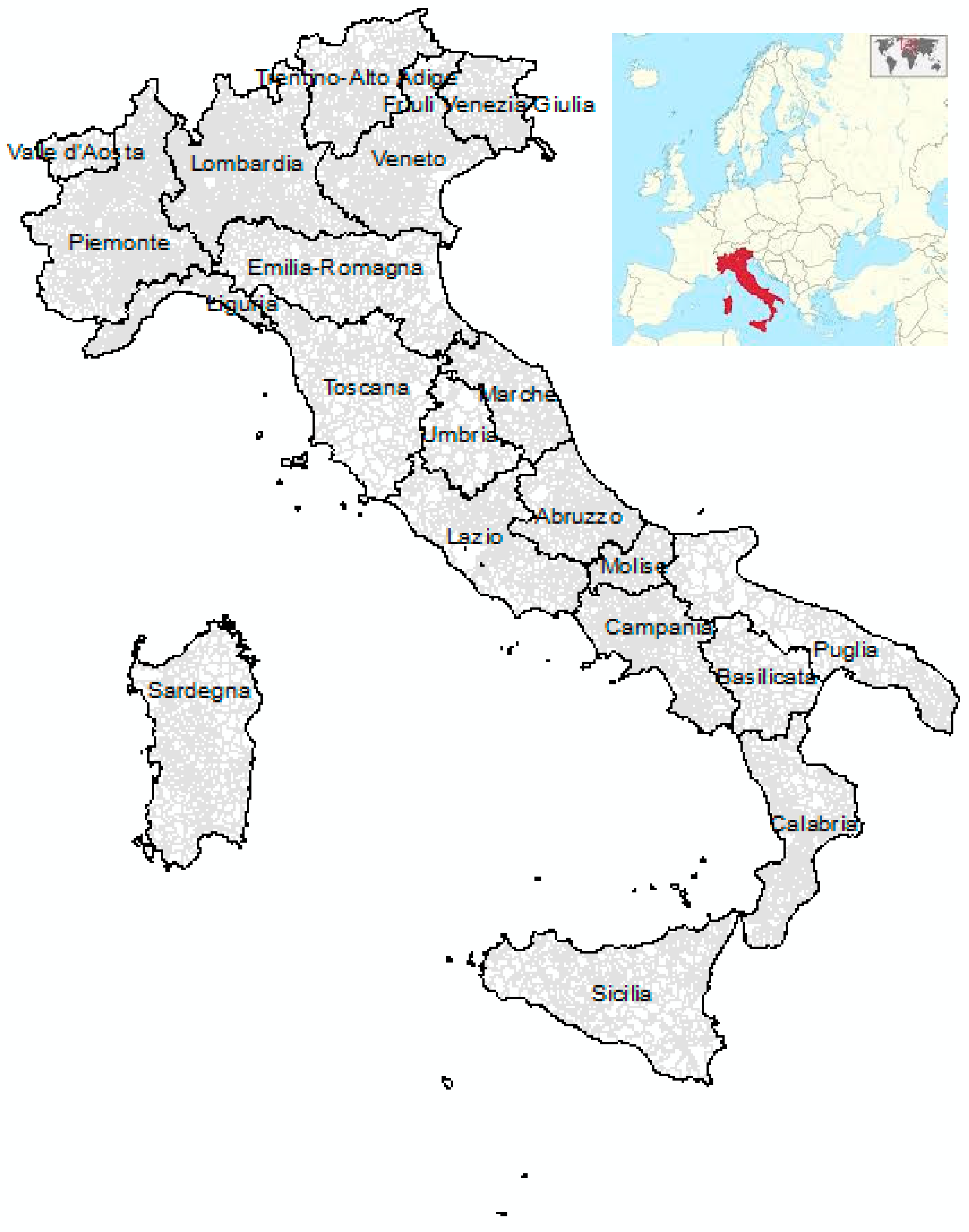The image showcases a detailed, hand-drawn map of Italy on a white background. The country and its regions are outlined in black, with dotted light gray and white sections differentiating each area. Prominent regions labeled in black text include Sicilia at the bottom, Calabria just above it, and other regions like Piemonte and Lombardia towards the top left. Additionally, the island of Sardegna is depicted separately from the mainland. In the upper right corner of the image, there is an inset map of Europe, where Italy is highlighted in red against a backdrop of yellow countries and light blue surrounding waters. This inset emphasizes Italy's location within Europe. The map precisely categorizes Italy's regions with clear, jagged lines, making it easy to distinguish each area.